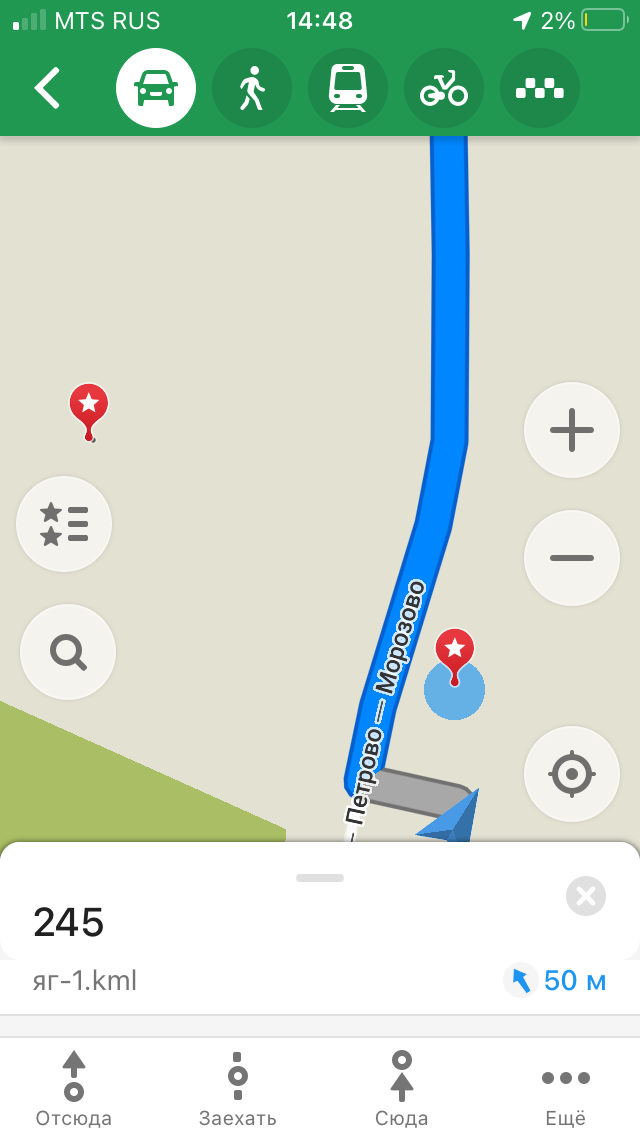The image is a screenshot of a phone displaying a map, likely from a navigation application such as Google Maps, with text predominantly in Russian. The phone screen shows a blue line indicating a car route with no signs of congestion. Notably, the map includes Russian labels, one of which is "Petrova Morozova," possibly a street name or area. The top of the screen highlights the MTS RUS service provider with a single cell signal bar, and the time displayed is 14:48 (2:48 p.m.). The phone's battery is critically low at 2%. Icons at the top depict different modes of transportation, reinforcing that the map is set for car navigation. Additionally, at the bottom of the screen, it indicates a distance of 45 kilometers and a partial data point of 50 meters.